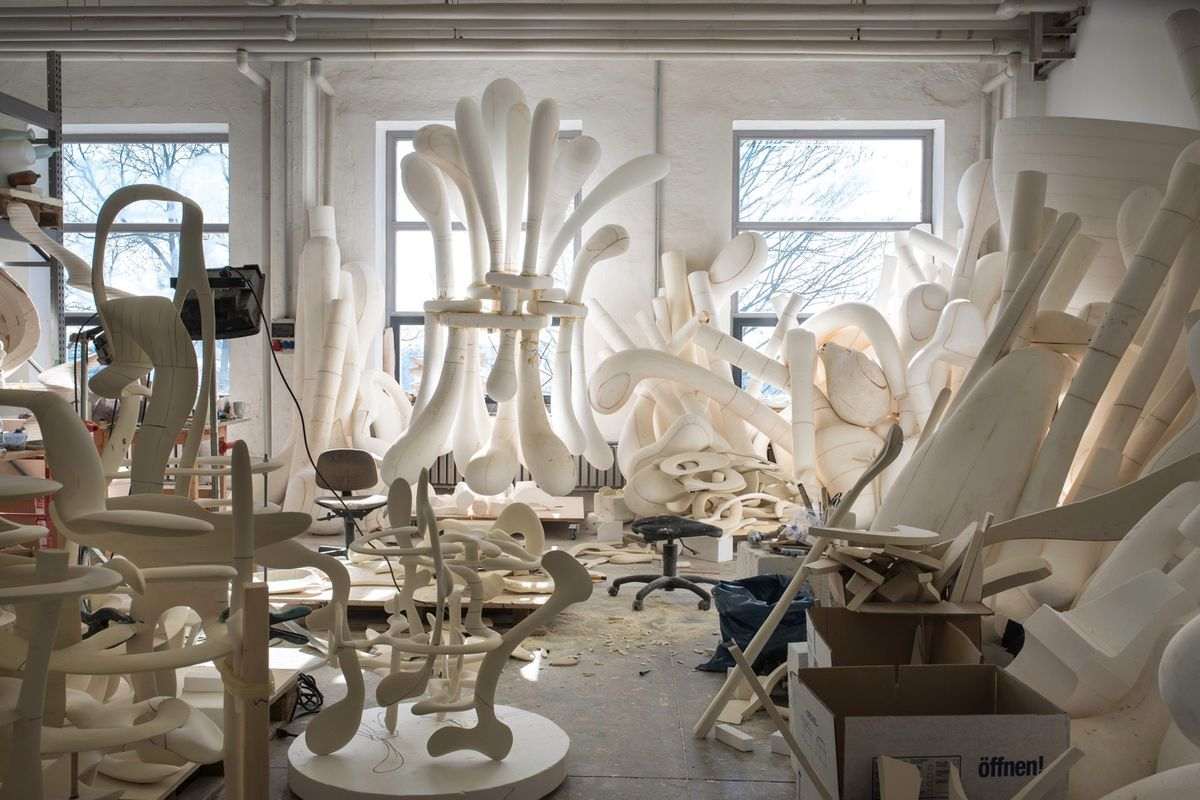The photo captures an intriguing scene inside what seems to be an artist’s studio, filled with a variety of white, oddly shaped sculptures. These sculptures, which are smooth and vaguely reminiscent of oversized Q-tips or bones, dominate the space in both clustered and individual arrangements. Some lean against the walls while others rest haphazardly across the floor, adding to the chaotic atmosphere. This mess is accentuated by the broken pieces of sculptures, empty cardboard boxes, and an abundance of debris including sawdust scattered across the floor. The room itself, likely an old warehouse or abandoned space repurposed as a studio, features three large vertical windows spaced evenly along one wall, bathing the room in natural light. Additional elements in the space include a black stool, a television monitor with wires trailing down, and white-painted pipes running along the ceiling, all contributing to a sense of ongoing creative activity amidst a somewhat disordered environment.